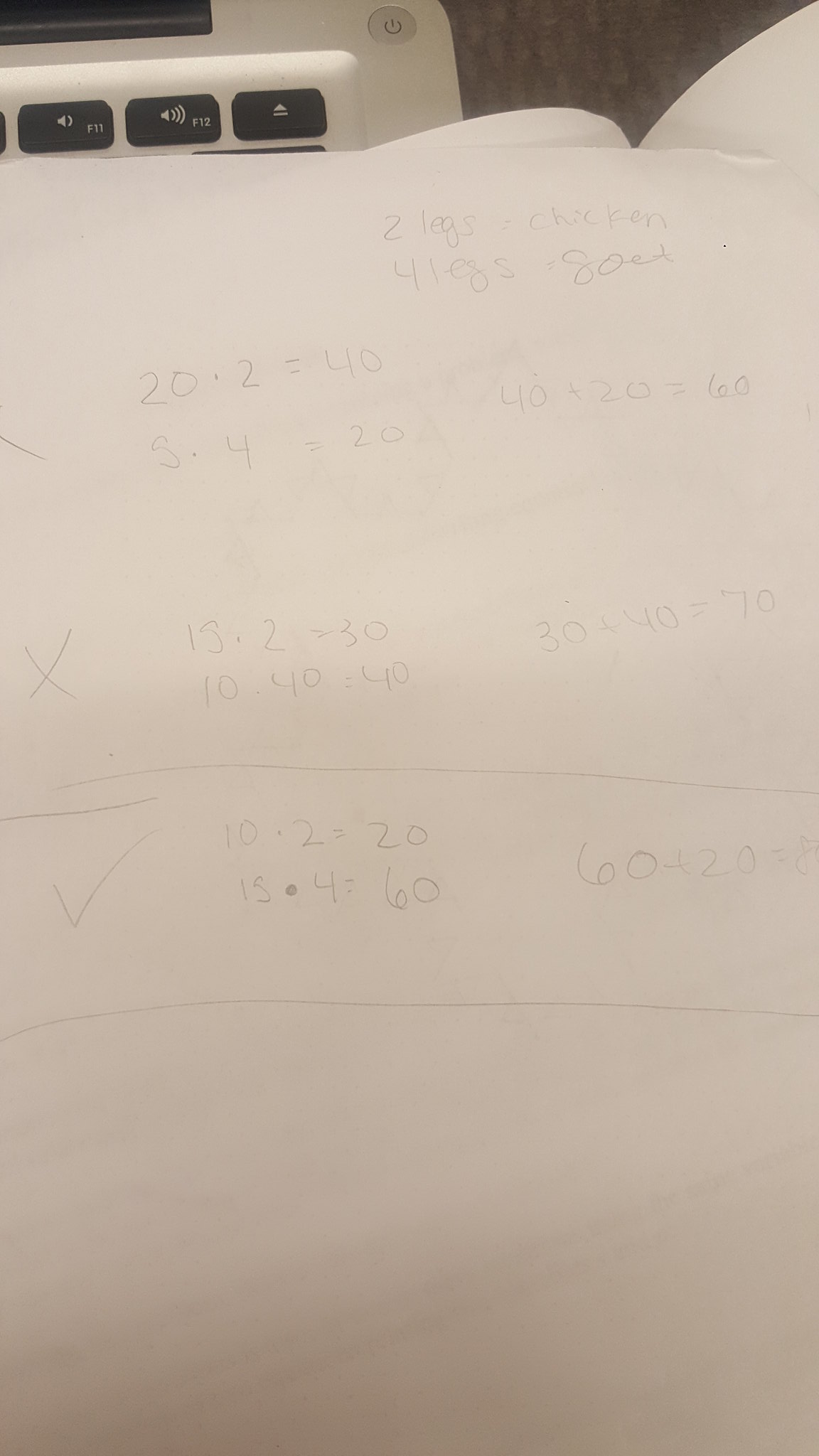In the image, a piece of paper is displayed containing handwritten math equations in pencil. The paper appears slightly cluttered and difficult to decipher at first glance. It begins with a note that reads "two legs equals chicken, four legs equals goat." Below this, there is a math equation written as "20 * 2 = 40" followed by "5 * 4 = 20." To the right side of these calculations, it states "40 + 20 = 60."

To the left of these notations, there are two X marks. The first X is accompanied by "15 * 2 = 30," and directly underneath, it says "10 * 4 = 40." Continuing downward, it adds "30 + 40 = 70" beside an X mark. 

Further down the page, there is a checkmark next to the final set of calculations, starting with "10 * 2 = 20" and "15 * 4 = 60," which sums up to "60 + 20 = 80." Despite a mistaken final result originally reading "60 + 20 = 8," missing the zero.

Across the paper, lines are drawn both above and below sections of the math equations. In the top left corner of the image, a laptop is partially visible, displaying only three keys.